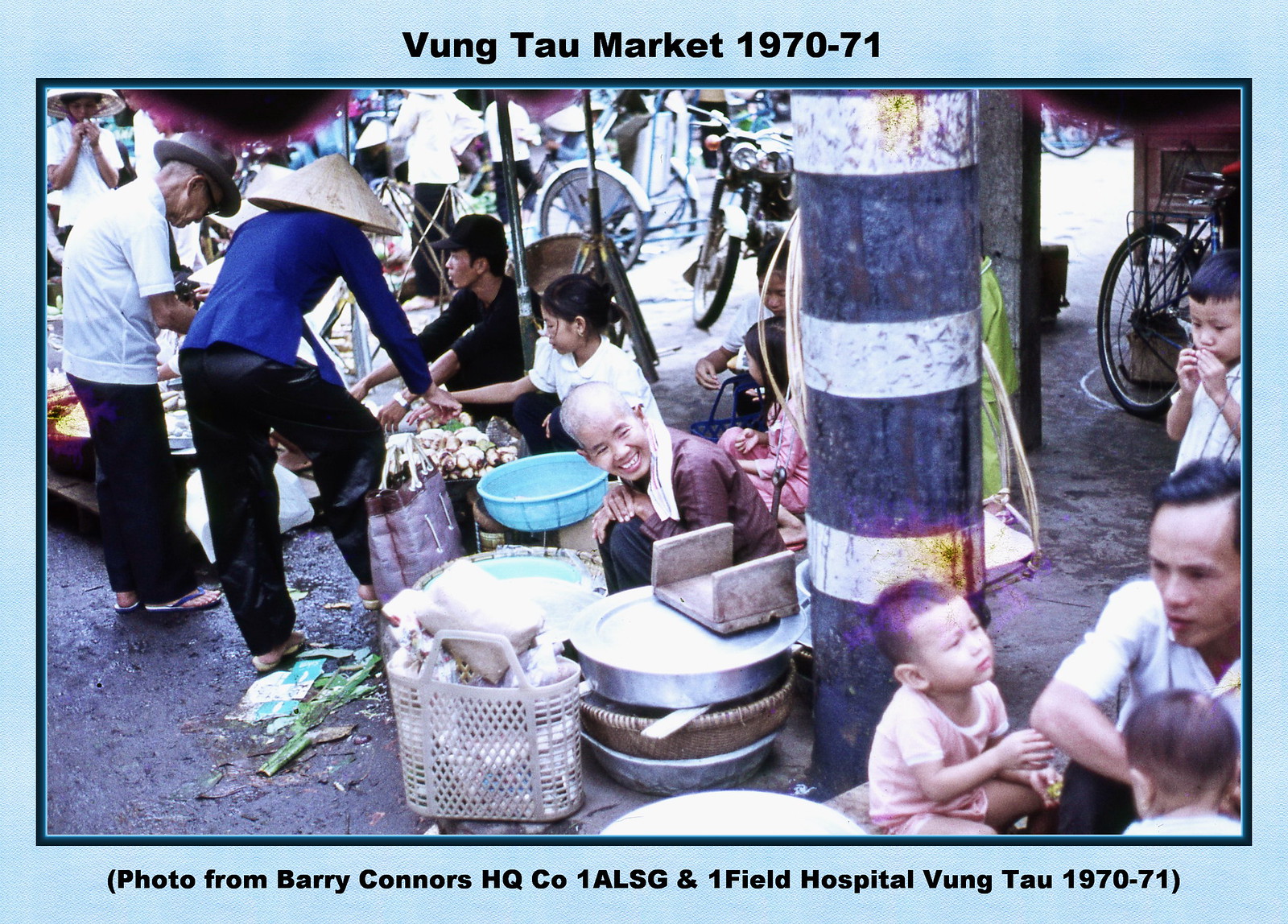This photograph captures a bustling market scene in Vung Tau, Southeast Asia, during 1970-71, as noted by the caption above the image which reads "Vung Tau Market, 1970 to 71" and attributes the photo to Barry Connors, HQ Colonel 1ALSG at Onefield Hospital Vung Tau. An Asian man, bald and smiling, sits at the center of the image, surrounded by various pots and receptacles, offering his wares while seated on the wet, dark brown mud ground. To the right, another Asian man is present with two children in front and another child standing behind him, partially obscured by a black and white striped post. On the left-hand side, additional vendors, some in rice paddy hats and flip-flops, are selling their produce to customers, who are dressed in a variety of clothing including blue and white shirts and black pants. In the background, a multitude of bicycles, motorcycles, and throngs of people add to the vibrant and lively atmosphere typical of a Southeast Asian market of the time.